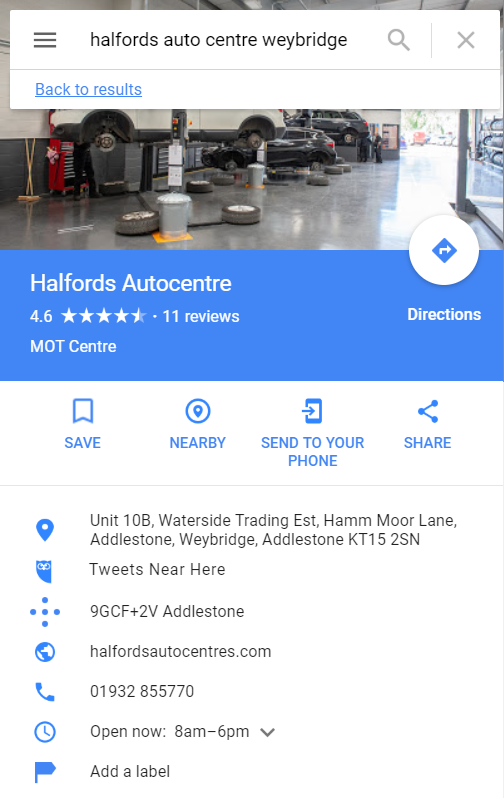Screenshot of a Google Maps search result for Halford's Auto Center in Weybridge.

The image showcases the Google Maps interface in a vertical portrait orientation as viewed on a smartphone. At the top, there's a search bar with "Halford's Auto Center Weybridge" entered. To the left of the search bar is a hamburger menu for additional options, and to the right, there is a magnifying glass icon for the search function and an 'X' button to clear the search.

Below the search bar, there's a hyperlink labeled "Back to results." Underneath it, a banner image depicts the interior of an auto garage. Below this, set against a blue background with white text, the location is identified as "Halford's Auto Center" with a 4.6-star rating based on 11 reviews, categorizing it as an MOT Center. Adjacent to this information, on the right side, is a directions button.

Further down, there are buttons labeled "Save," "Nearby," "Send to your phone," and "Share."

Detailed information follows below these buttons:
- **Address:** Unit 10B, Waterside Trading Establishment, Hamm Moor Lane, Addlestone, Weybridge, Addlestone, KT15 2SN.
- Additional location info includes a Plus Code: 9GCF+2V Addlestone.
- **Website:** halfordsautocentres.com
- **Phone Number:** 01932 855770
- **Opening Hours:** Currently open, from 8 a.m. to 6 p.m.
- There is also an option to add a label to this entry with a flag icon.

The clean and detailed description offers a clear understanding of the screenshot's content as presented on an iPhone.